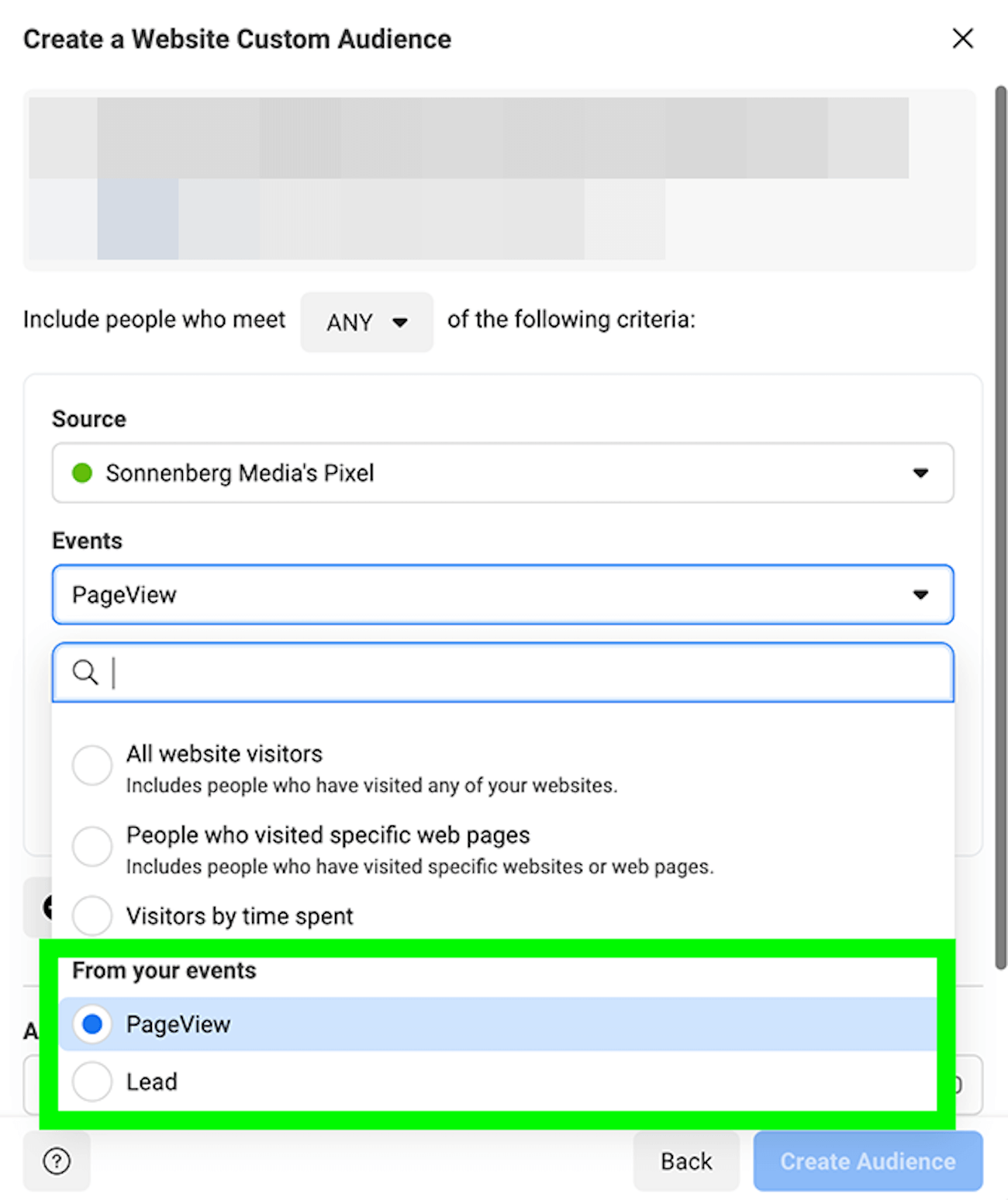Screenshot of a website labeled "Create a Website Custom Audience." The interface predominantly features a black-and-white color scheme with blue and green highlights accentuating certain elements. At the top of the screenshot, the title "Create a Custom Website Audience" is displayed prominently.

Below the title, there is a grayed-out section that appears to be obfuscated for privacy reasons. Directly beneath this gray area, the text "Include people who meet any of the following criteria" is shown, indicating that users can select specific criteria for their audience.

The next section includes a mention of "Source: Sonnenberg's Media Pixel," suggestive of a tracking pixel used for collecting website data. This section is interactive, allowing users to potentially select or modify the source. There is a dropdown or expandable menu labeled "Events," which likely provides additional options for criteria selection.

Further down, there are options for targeting specific types of website visitors. These options include:
- "All Website Visitors": Targets individuals who have visited any of your websites, possibly aggregating data across multiple sites.
- "People who visited specific web pages": Focuses on users who have viewed particular pages.
- "Visitors by time spent": Allows for the segmentation of audience based on the duration of their visits.

The screenshot appears to be part of an advanced targeting interface designed to help users build custom audiences based on detailed web traffic data.